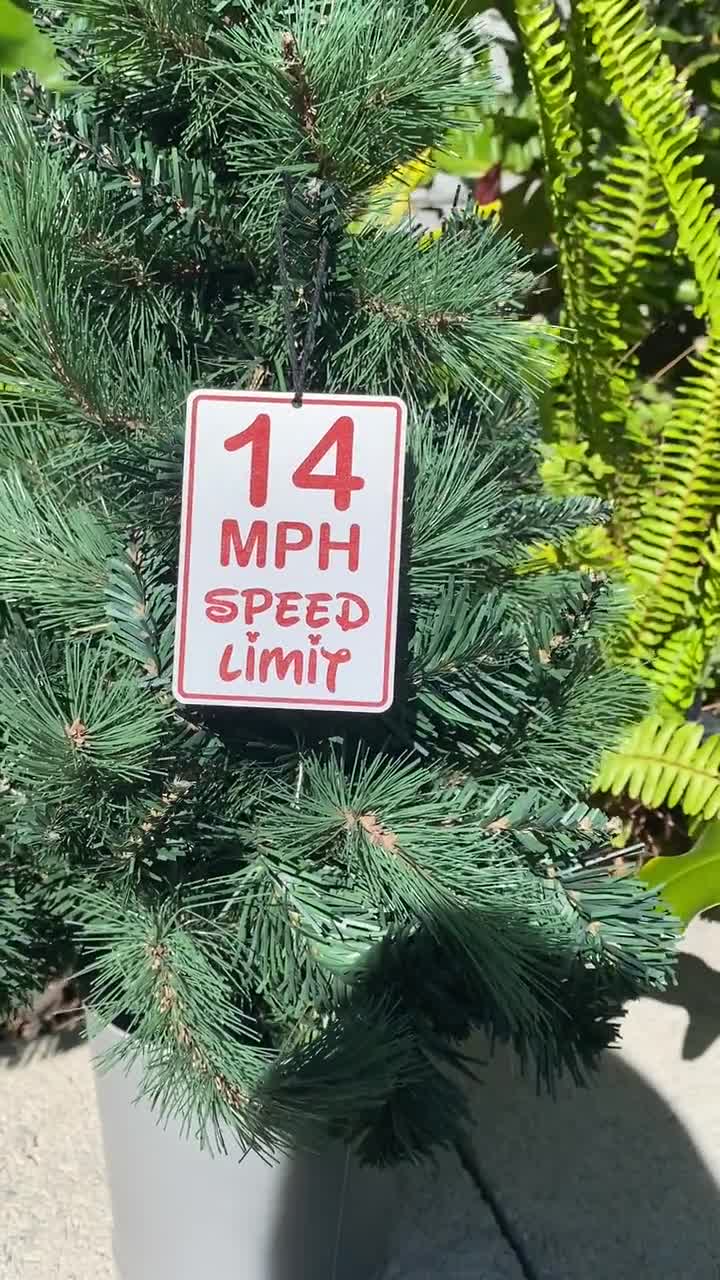The image features a portrait-oriented photograph, roughly twice as tall as it is wide, set outdoors under natural sunlight coming from behind the viewer. Dominating the scene is a small, dark green pine tree, reminiscent of a tiny Christmas tree, positioned in a gray potted planter on a gray, cracked sidewalk. The pine tree’s needle-like branches occupy much of the frame, with a secondary, out-of-focus tree-like object showing lighter green leaves in the background. Attached to the tree is a distinctive, small white sign with a red border and red lettering, stating "14 MPH" in a standard font and "speed limit" in a dripping effect. The sign also has Mickey Mouse-shaped dots over the letter 'I's, possibly hinting at a Disney-themed setting. A shadow, most likely of the photographer, is cast across the sidewalk and partially on the tree, appearing on the right third of the image.